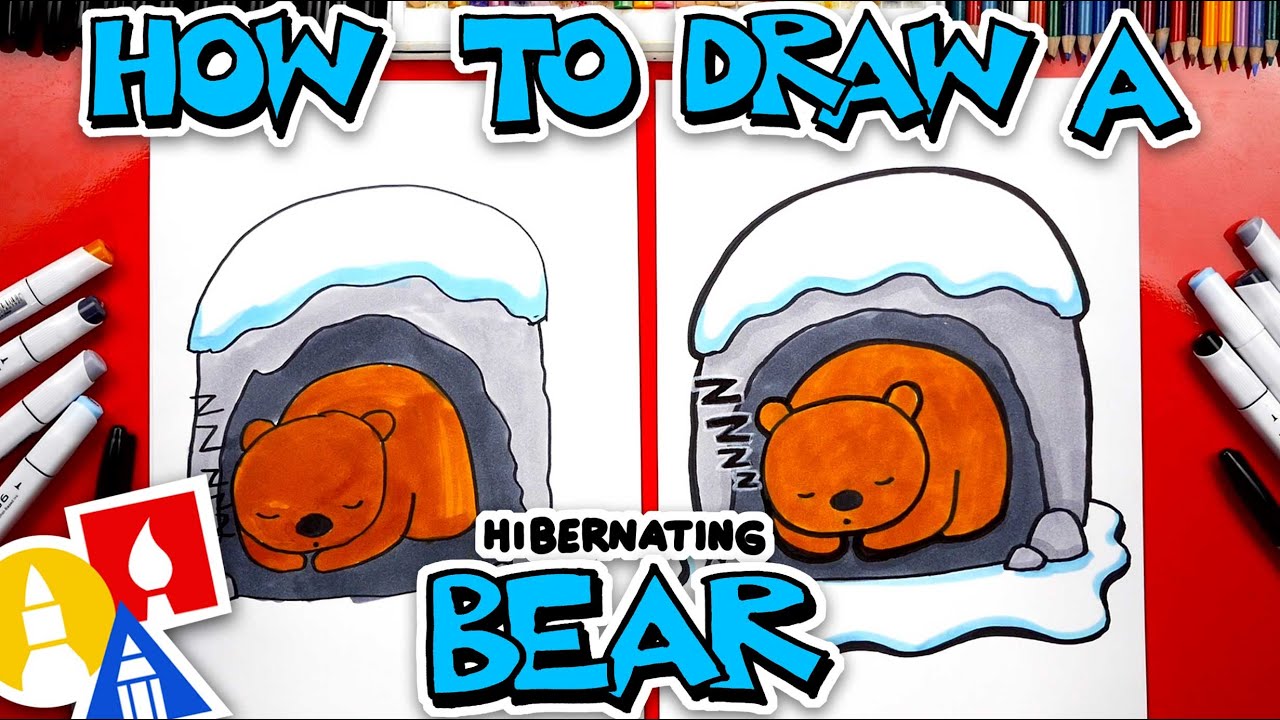The image is a detailed instructional guide on how to draw a hibernating bear. This guide features two side-by-side cartoon panels of a brown bear, eyes closed and head resting on its paw in a snow-covered cave. The bear in the left panel appears less finished, while the one on the right is more refined. At the top of the image, in light blue all-caps text with a black outline, it reads, "HOW TO DRAW A," followed by "HIBERNATING" in smaller all-caps text, and "BEAR" beneath it. The image is set on a red table with various colored markers, colored pencils in the corners, and other drawing tools on either side. A distinctive watermark featuring a marker in a yellow circle, a paintbrush in a red square, and a pencil in a blue triangle is located in the bottom left-hand corner. The primary colors in the image include red, white, blue, light blue, gray, dark gray, sky blue, orange, and orange-brown.